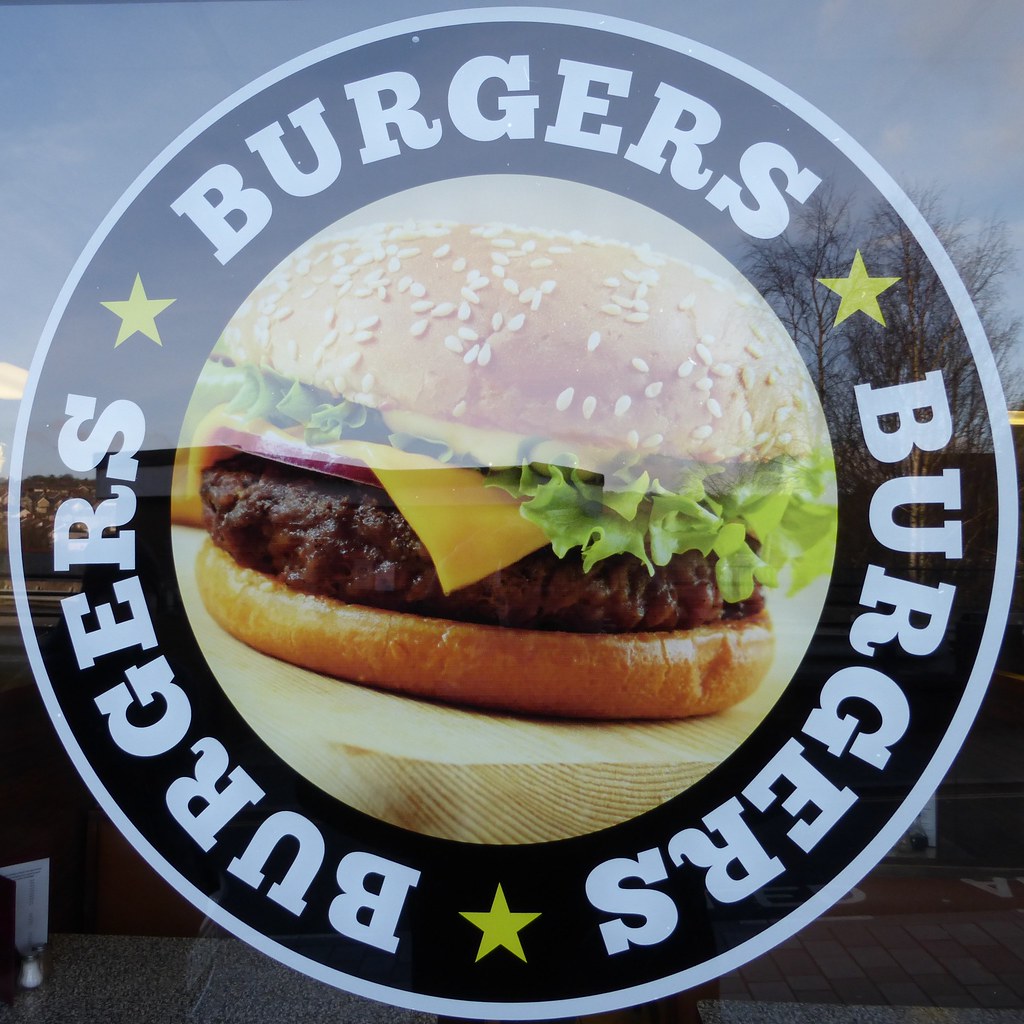The image is a detailed photograph of a circular sticker placed on the inside of a restaurant window. The sticker, featuring a white border and an outer black ring, prominently displays the word "BURGERS" in capital letters three times, each separated by a yellow star. At the center of the sticker is a vivid, close-up photograph of a burger with a sesame seed bun. The burger includes layers of cheese, leafy lettuce, a slice of red onion, and a meat patty, all seemingly placed on a wooden table. Reflected on the window are clear elements of the outdoor scenery, including blue skies with a few clouds, a tree, and a walkway. The atmospheric reflection adds a visual depth to the image, tying together the exterior backdrop and the enticing close-up of the burger, suggesting the interior setting is indeed a burger-focused restaurant.